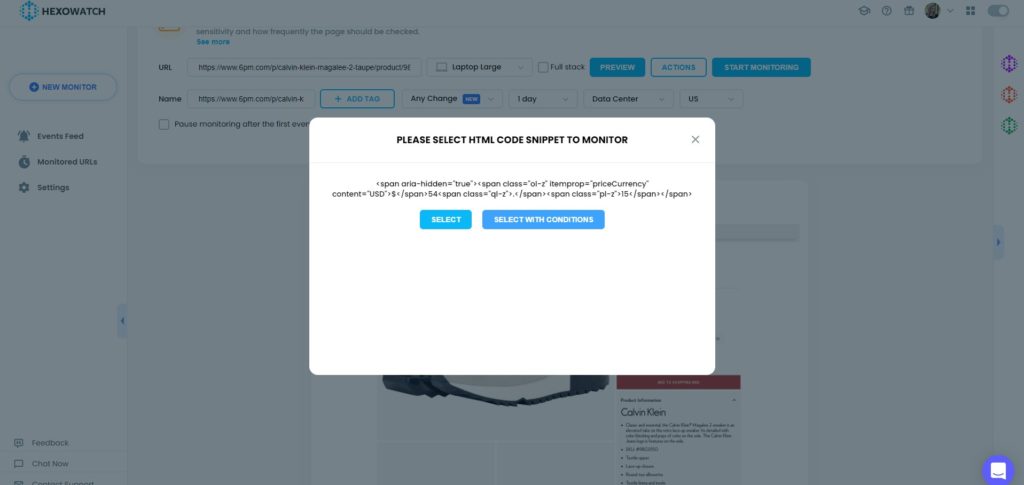The image is a screenshot displaying an open web page that has been grayed out due to an overlayed pop-up menu. The central pop-up menu features a clean, white background with a header in black font reading, "Please select HTML code snippet to monitor." Directly below the header is a horizontal black line, followed by an HTML code snippet also in black font. Towards the bottom of the pop-up, there are two blue rectangle buttons; the one on the left has white text that says "Select," and the one on the right reads "Select with conditions."

In the background, the grayed-out web page is identified at the top with the title "HexoWatch" in black font. To the left of the title is a stylized logo consisting of a white "H" encircled by blue dots. On the upper right corner of the page, there are three gray icons: a question mark inside a gray circle, a small gift box, and what appears to be a user's profile picture, though the latter is too small to discern clearly. 

This detailed context provides a comprehensive understanding of the interface and elements visible in the screenshot.